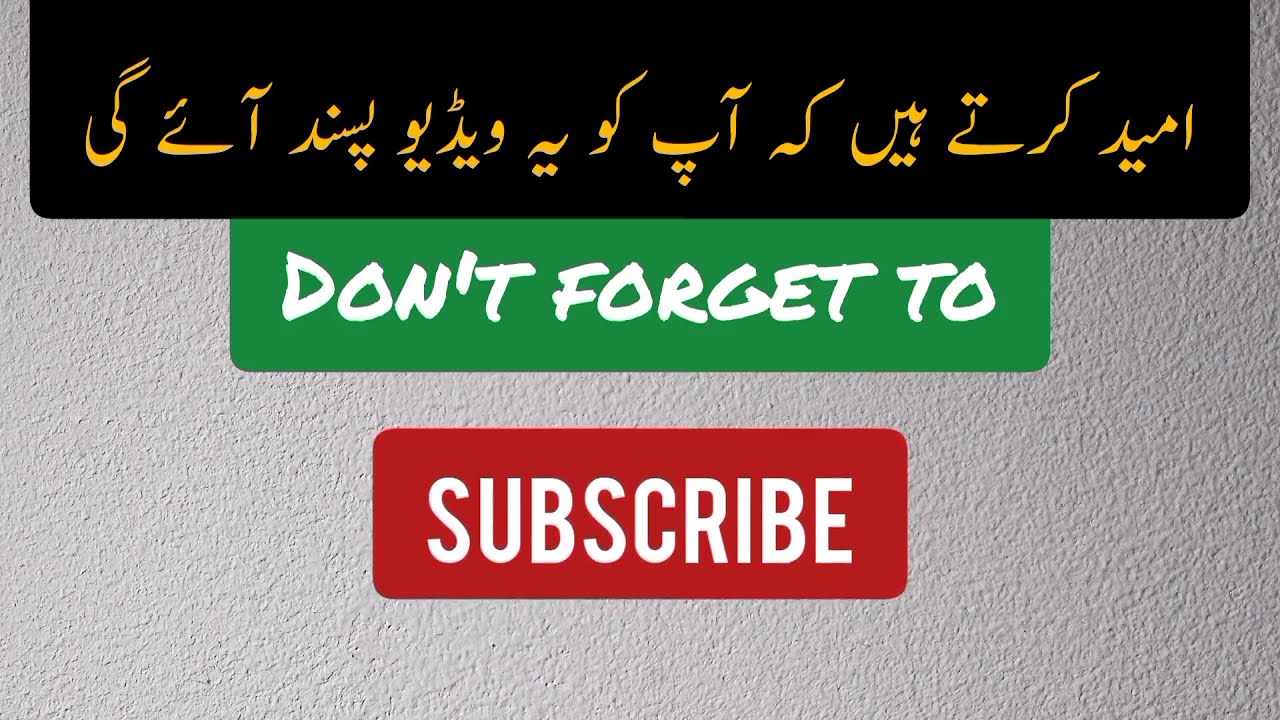The image features a gray, textured background resembling a rough, possibly photographic depiction of a wall. This background showcases constant bumps and divots, giving it a tactile, uneven surface. Dominating the top section of the image, a black stripe spans almost the entire width, containing gold characters that appear to be in a Middle Eastern or Asian script. Directly below this is a green stripe, also stretching almost the entire width, which displays the phrase "DON'T FORGET TO" in thick, white, uppercase letters. Finally, positioned below and centered relative to the green stripe is a red rectangle, which prominently features the word "SUBSCRIBE" in bold, uppercase white letters.